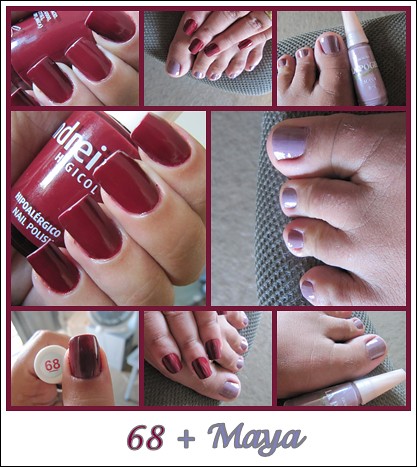The image appears to be a detailed nail polish advertisement, featuring a photo montage of eight photographs showcasing hands and feet with painted nails. The montage emphasizes a contrast between two nail polish colors: a deep burgundy for the fingernails and a light lavender for the toenails. At the center of the composition are two prominent images; one shows a person’s hands proudly displaying their freshly manicured fingernails while holding the corresponding nail polish bottle, and the other shows a foot with chubby toes and a distinctive curve in the big toe, resting on a gray surface, highlighting the everyday nature of the model. Additional smaller images surround these central photos, providing various perspectives of the painted nails. The montage is bordered in burgundy, adding a cohesive frame to the layout. At the bottom of the picture, the text "68 plus Maya" is written in gray, alongside a note indicating the polish is hypoallergenic, though the specific brand name is not visible. The overall presentation suggests a promotion of the nail polish's versatility and appeal for everyday use, showcasing the elegance of the burgundy for fingernails and the softness of the lavender for toenails.